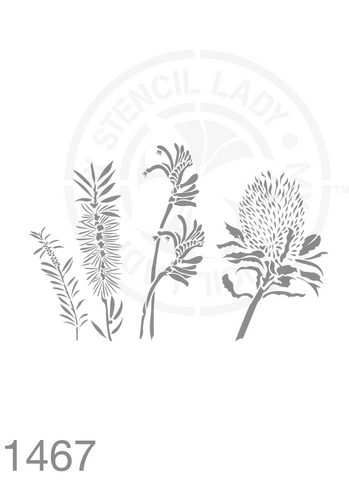This monochrome image predominantly features the detailed outlines of various plants, likely depicting a mix of weeds, flowers, and grasses, arranged across a white background. The plants, four in total and drawn in various shades of gray, extend vertically with each featuring unique characteristics. The first plant on the left is delicate with thin leaves, while the second plant is taller and more prickly. The third plant consists of two intertwined vines adorned with thicker leaves, and the fourth plant has more pronounced prickly leaves with a prominent, flowery top. These botanical illustrations are overlaid on a rounded, concentric logo inscribed with "Stencil Lady" in lighter gray, though some of the finer details of the logo remain obscured by the plants. In the bottom left corner, the number "1467" appears in the same gray hue as the plants, further blending into the artwork. The overall composition seems to highlight stencil work, showcasing the intricate, fibrous textures and varying stem lengths of each plant in a style that is likely digitally rendered.